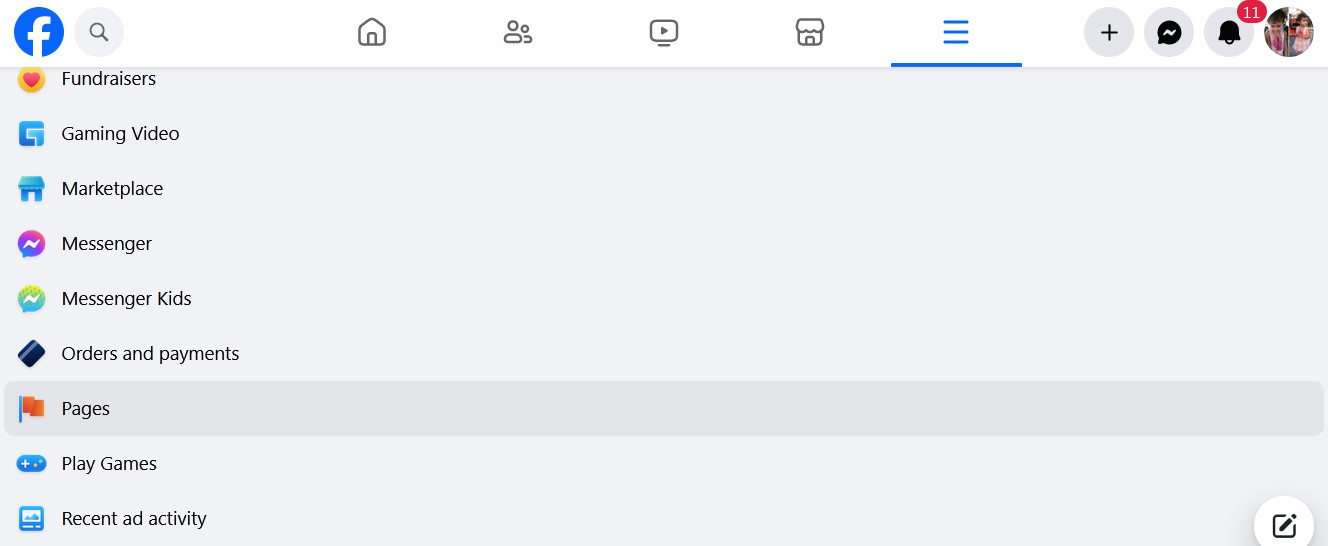The image showcases the Facebook app interface. At the top left, the Facebook icon is prominently displayed, next to which sits a search icon. The interface is primarily off-white with black text. Moving horizontally to the right from the search icon, there is a sequence of icons: a home icon, an icon depicting two people, a videos icon, a Facebook Marketplace icon, and a set of three horizontal bars (which is highlighted in blue, indicating it’s selected). Next to these icons, there is a plus sign, the messenger icon, a notifications icon with a red badge showing the number 11, and finally, a profile icon.

Beneath this main menu bar, there is a vertical list of various Facebook sections: 'Fundraisers' (illustrated with a yellow circle containing a red heart), 'Gaming Video' (marked with a 'G'), 'Marketplace' (displayed as a shop icon), 'Messenger' (the well-known messenger app icon in purple), 'Messenger Kids' (the messenger app icon in green), 'Orders and Payments' (depicted with a credit card icon), 'Pages' (highlighted with an orange flag since it is the currently selected section), 'Play Games', and 'Recent Ad Activity'. Each of these sections is accompanied by a relevant icon. Additionally, a small ad icon is visible in the bottom right corner of the list.